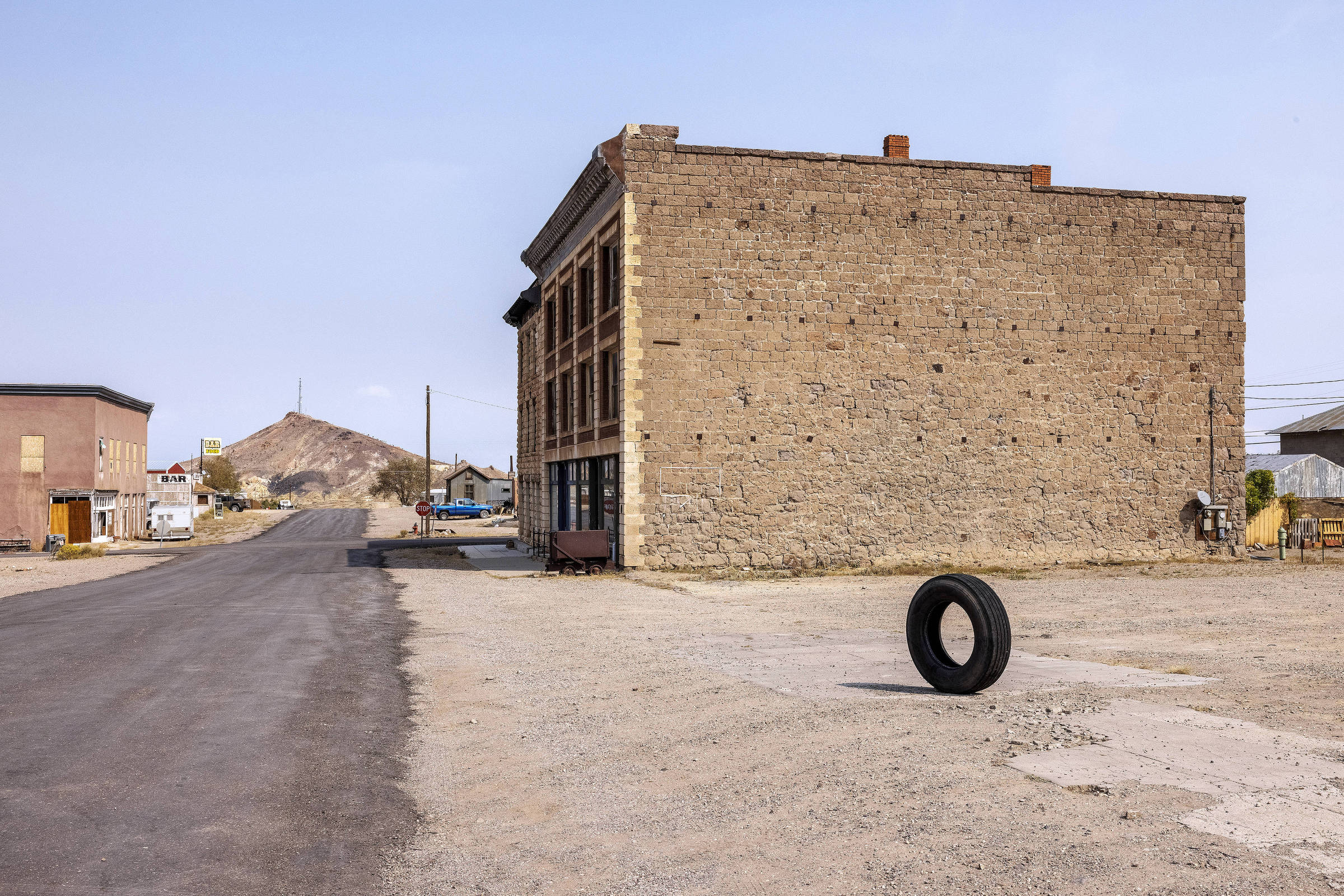The image captures a desolate scene outside a large stone building, characteristic of an older, possibly abandoned property. The building, constructed from stone bricks, stands prominently on the right side of a small four-way intersection. Adjacent to it is a gravel parking lot, where a lone tire, devoid of its rim, stands upright at its center. 

A paved black road runs along the left side of the photo, disappearing into the distance, typical of a small town with undefined edges. In the background, a mound of dirt is visible, accessible by a road leading directly to it. This road is flanked by a small building or shed and a blue truck. Across the street from the stone building and parking lot is a smaller, two-story building with boarded-up windows, both on its top and bottom floors.

Further in the distance to the left, another small building sports a sign that reads "Bar," enhancing the sense of an isolated, almost forgotten place. Topping off this liminal scene, a large hill rises in the background, crowned with what appears to be a radio or cell tower, completing the eerie and vacant atmosphere of the photograph.